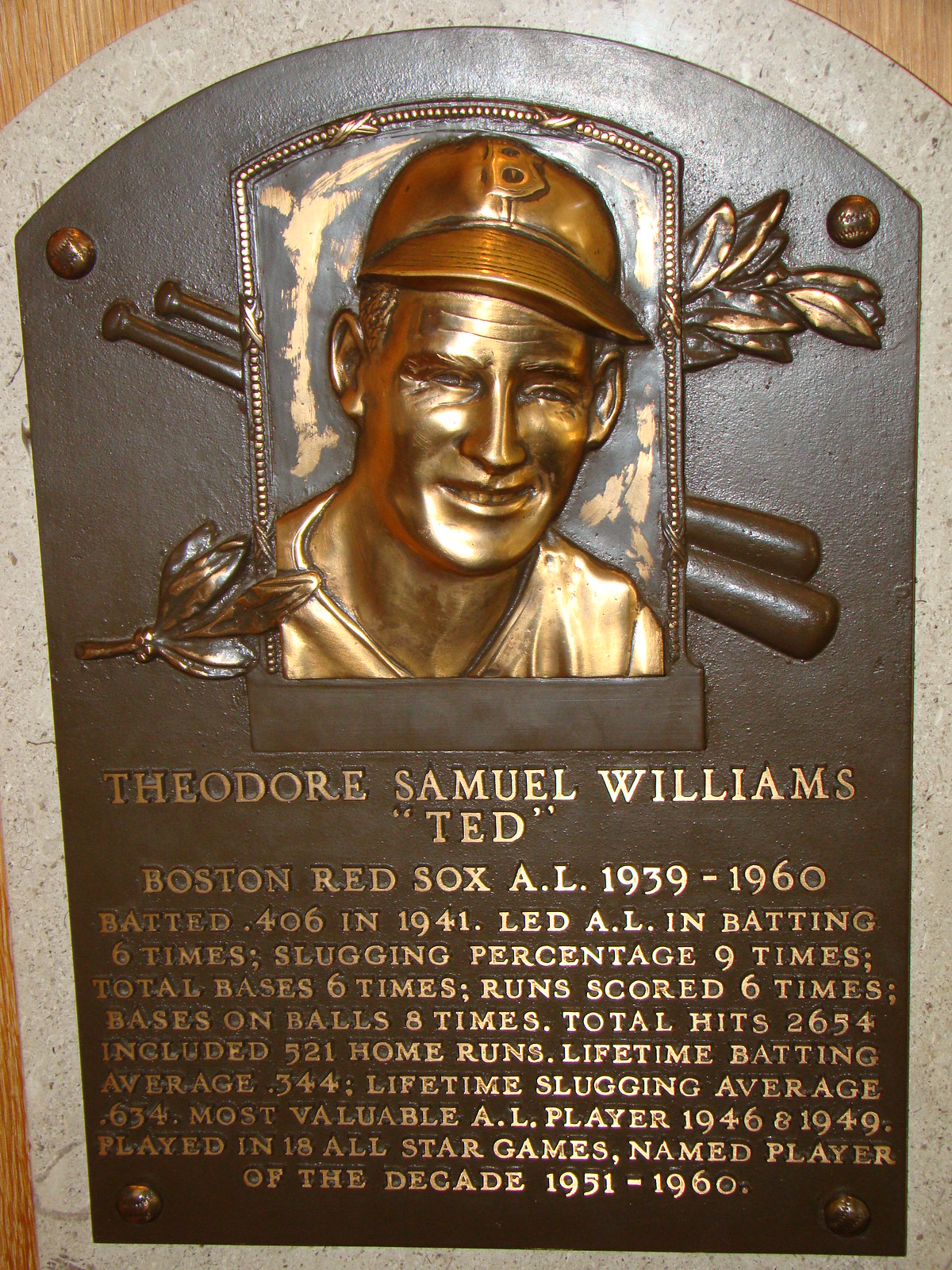This image showcases a memorial plaque dedicated to the revered baseball player Theodore Samuel Williams, popularly known as "Ted" Williams. The plaque's design features a curved top with straight side and bottom borders in light gray, and its main background is dark green. The centerpiece includes an embossed golden likeness of Ted Williams, smiling and wearing a baseball cap and jersey, designed with intricate plant leaf patterns and visible screws securing the plaque at the top and bottom. The detailed golden inscription highlights his illustrious career with the Boston Red Sox from 1939 to 1960. The text commemorates his achievements, including leading the American League in batting six times, slugging percentage nine times, and total bases six times. Additional accolades note his .406 batting average in 1941, scoring six times, accumulating 2,654 hits including 521 home runs, maintaining a lifetime batting average of .344, and a slugging average of .634. He was named the American League's Most Valuable Player in 1946 and 1949, participated in 18 All-Star games, and earned the title Player of the Decade for 1951-1960.